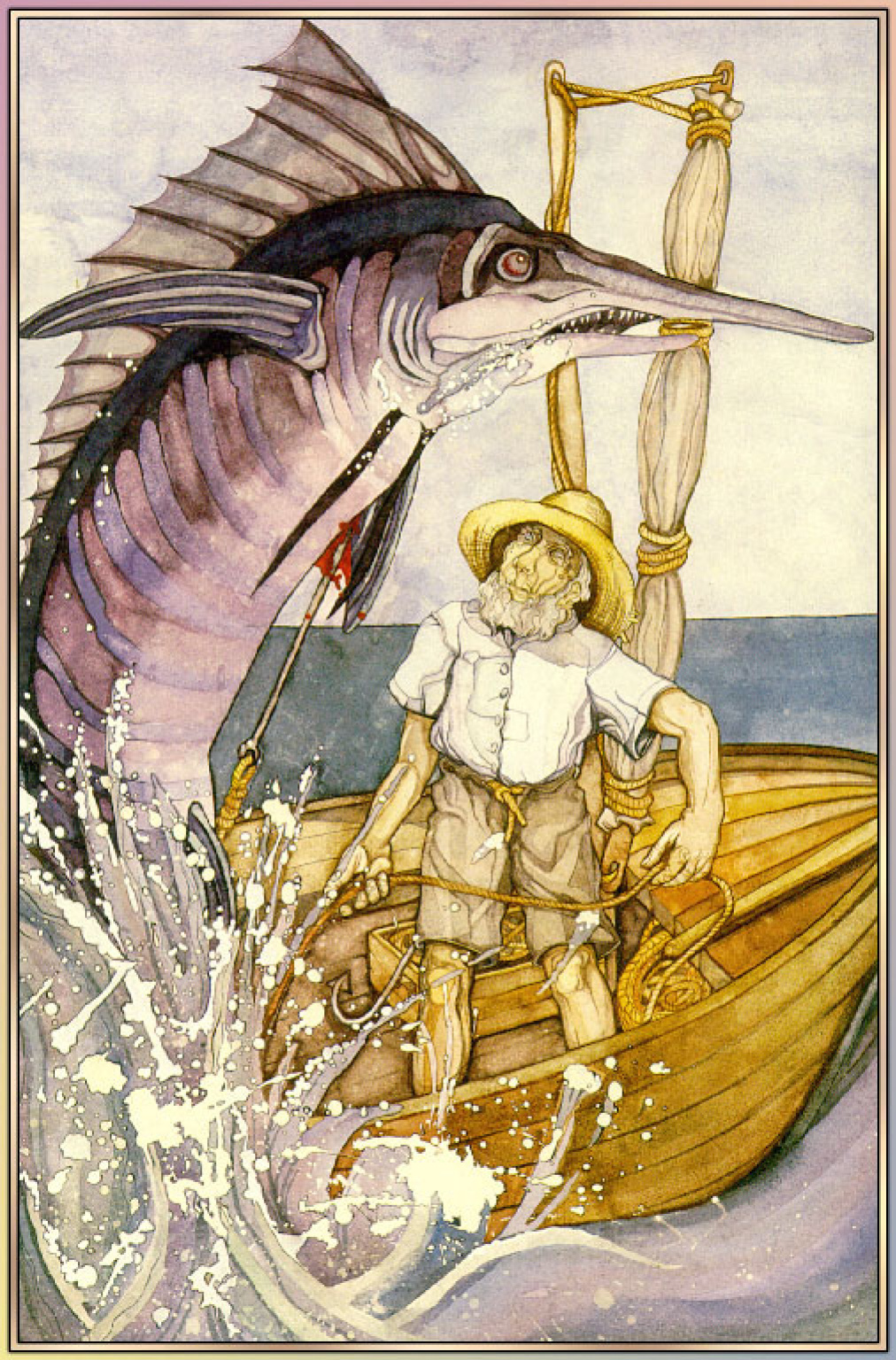The image is an old-fashioned, storybook-like illustration set in a vertical rectangle depicting an elderly fisherman with a thick gray beard in a very small, unpainted wooden sailboat. He is wearing a straw hat, a simple white button-up shirt, and beige shorts held up by a rope belt. The boat has a tied-up mast, and a bit of fishing gear and a box can be seen inside it. The fisherman holds a rope in his hand and is gazing up in awe at an enormous fish, possibly a marlin or sailfish, that is dramatically emerging from the water with a huge splash on the left side of the scene. The fish, with its colorful hues of pinks, blues, browns, and grays, arches magnificently over the entire frame, seemingly poised to overtake the tiny vessel. The background features a sliver of the blue-gray sea and some clouds, enhancing the dramatic tension of this captivating moment. The scene evokes a sense of adventure reminiscent of classic tales like "Call me Ishmael" and "The Old Man and the Sea."